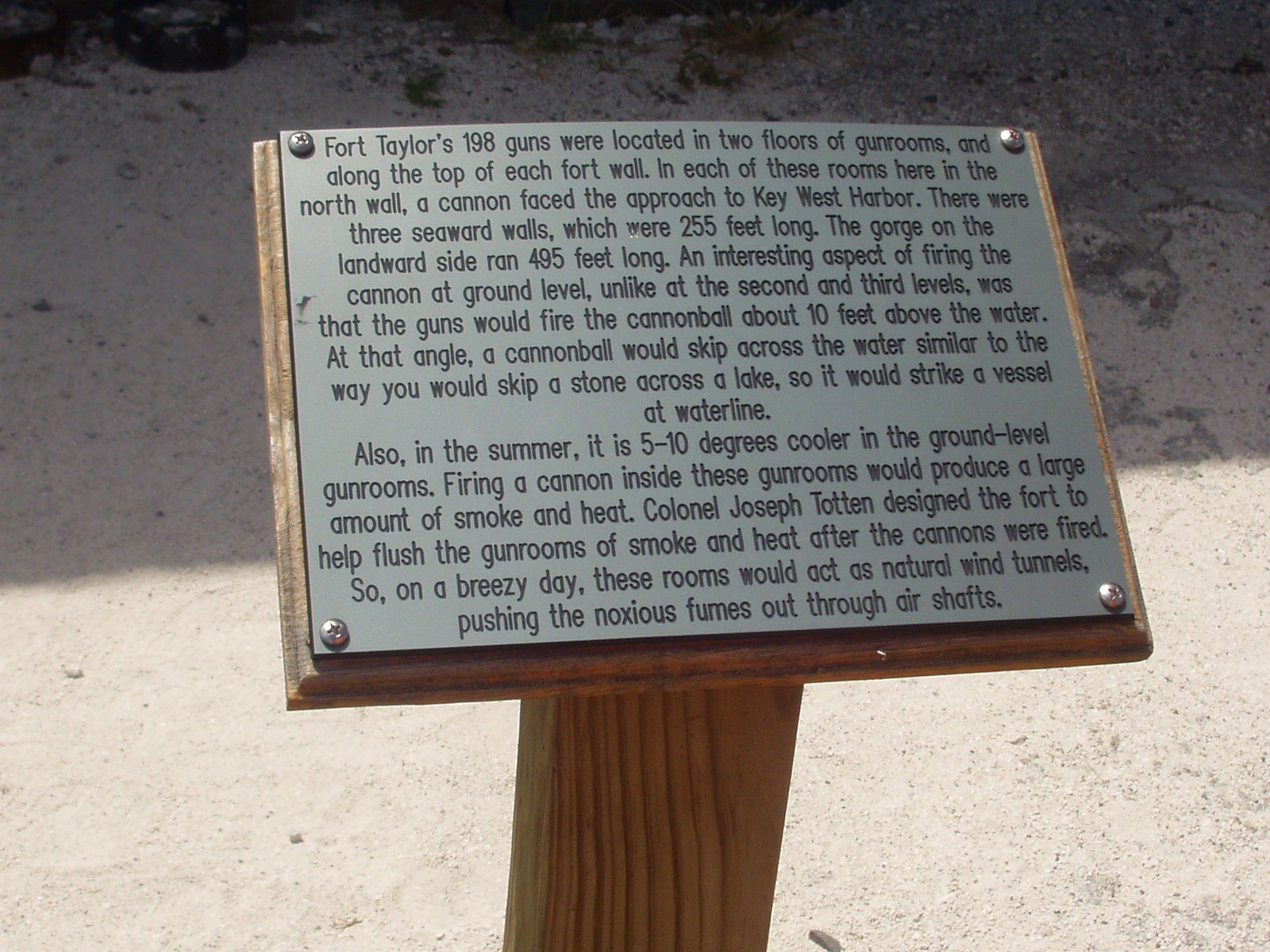The image showcases a detailed photograph of a historical plaque mounted on a square wooden base affixed to a plain wooden post, which appears to be embedded either in sandy or cement substrate. Positioned centrally amidst some rocks visible towards the top, the sign provides intricate historical information about Fort Taylor. The metal plaque, secured with screws at all four corners, bears black text that reads: "Fort Taylor's 198 guns were located in two floors of gun rooms and along the top of each fort wall. In each of these rooms, here in the north wall, a cannon faced the approach to Key West Harbor. There were three seaward walls, which were 255 feet long, while the gorge on the landward side extended 495 feet. An interesting aspect of firing the cannon at ground level, unlike at the second and third levels, was that the guns would fire the cannonball about 10 feet above the water, causing it to skip across the surface and strike vessels at the waterline. Additionally, these gun rooms, 5 to 10 degrees cooler in summer, contained design features by Colonel Joseph Totten to expel smoke and heat via natural wind tunnels on breezy days.” The scene depicted is notably outdoor, likely in the middle of a sunny day at a beachside location.